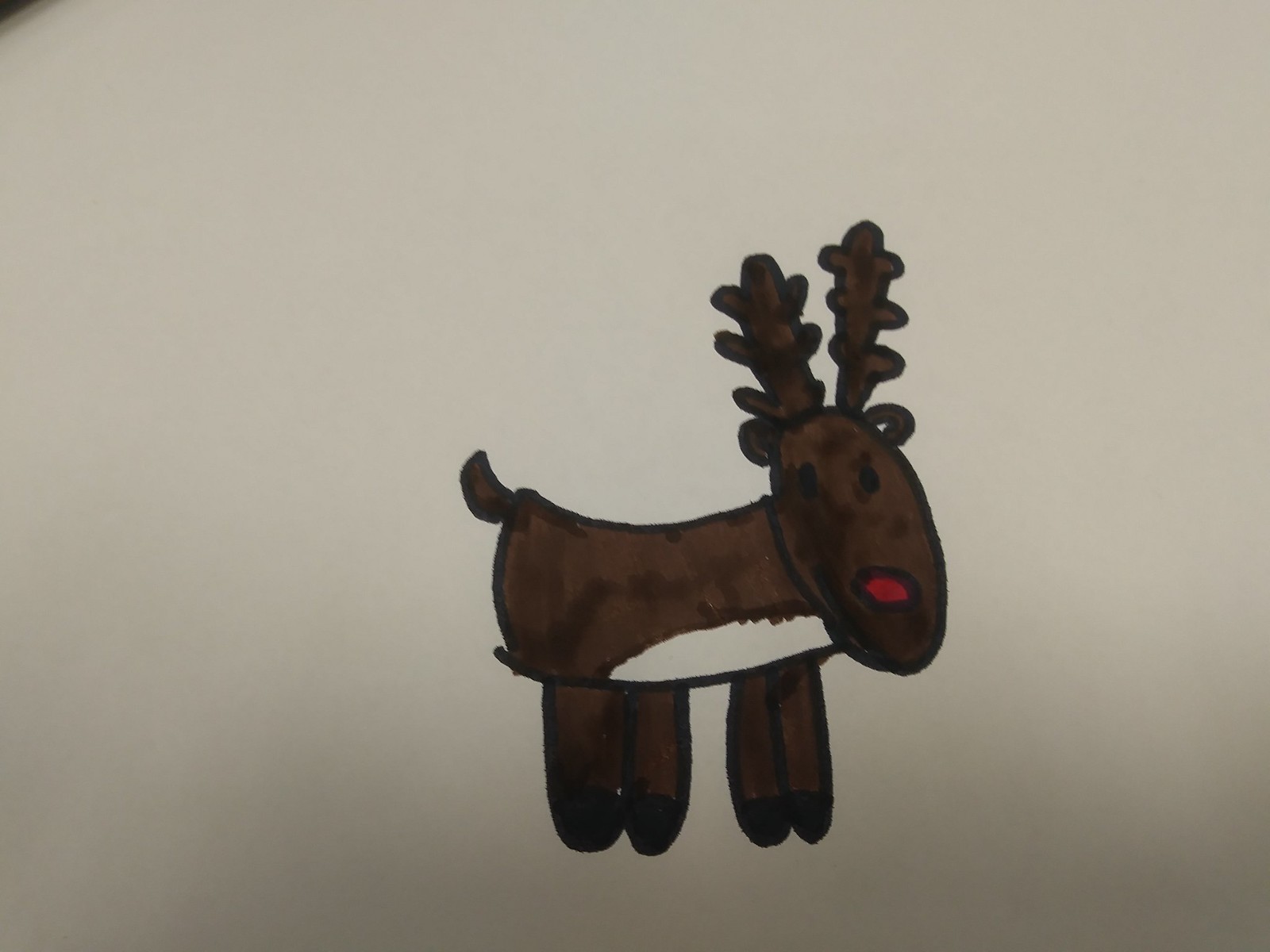The image features a simple, childlike drawing of a reindeer, done in marker, on a plain off-white or tan piece of paper. The reindeer’s body is oriented toward the three o'clock position while its head faces the viewer. The body is shaped like a sideways rectangle with a white belly and four elongated, arch-like legs extending downward. It has a brown tail and oval-shaped head adorned with two semicircular ears, one of which has a hint of white. The reindeer sports two antlers, dark almost indistinguishable eyes, and a vibrant red nose, but no mouth. The sketch is colored using brown marker for the body, black for the outline, and some red for the nose. It's an extreme close-up, causing the face to appear quite dark, and the drawing isn't well lit, leaving minimal details visible beyond the reindeer's basic features.